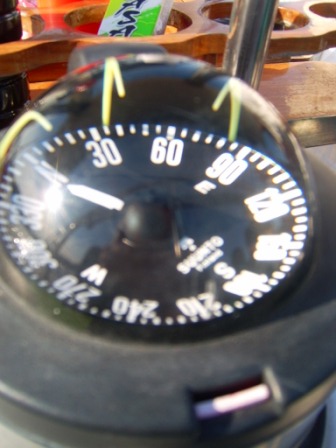The image features a vintage car compass, designed to be placed on a dashboard. The compass has a spherical shape, with a transparent glass ball containing compass markings that float on a liquid. The compass displays cardinal directions—north, south, east, and west—accompanied by degree markings. To the right of north are markings for 30, 60, and 90 degrees (east); south is marked by 120, 150, and 180 degrees; west shows 210, 240, and 270 degrees; and the degrees loop back to 300, 330, and north again. An arrow is currently pointing towards the north. The compass appears to be mountable on a car dashboard, likely with a suction cup and a release button for easy removal.

However, the setting in the image is not a car interior but a restaurant or eatery. The background features a wooden board with cutouts designed to hold cups. A green and white drink container labeled "ASA" is visible in one of the cutouts, enhancing the casual dining atmosphere.